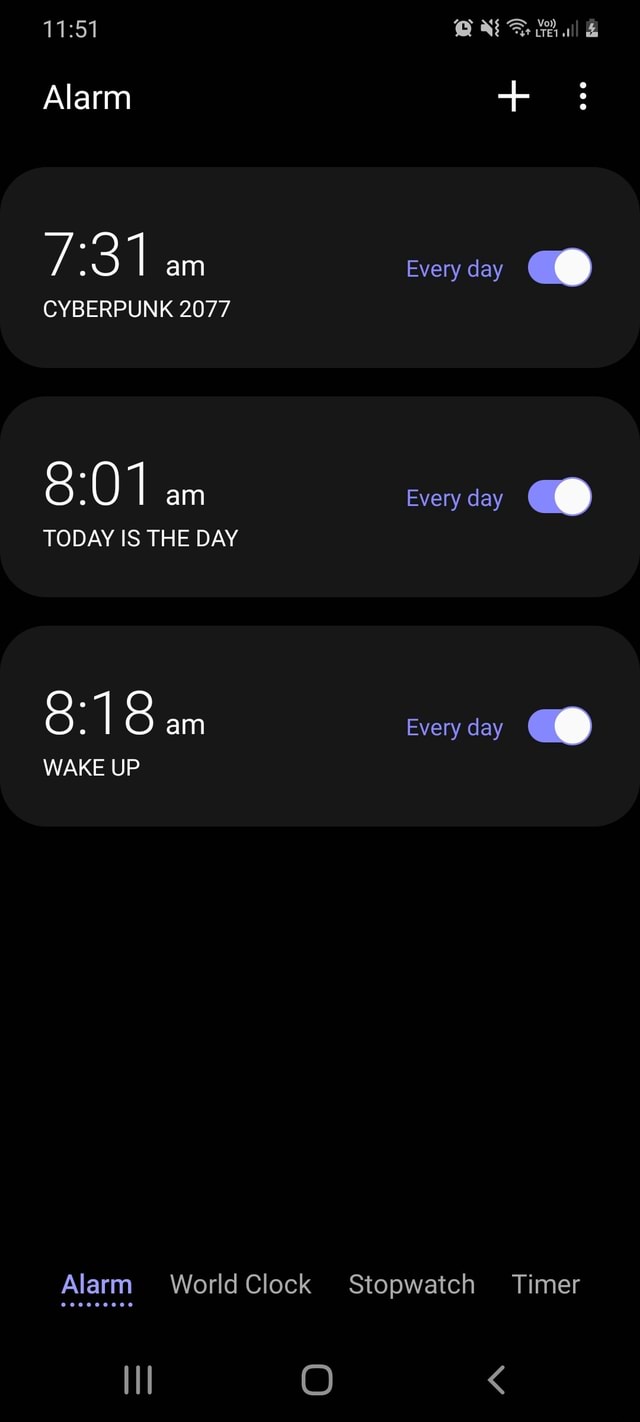This vertical screenshot captures the alarm-setting interface on a smartphone, featuring a black background. At the top, the current time, 11:51, is displayed in the upper left-hand corner, while the upper right corner shows system icons. Beneath the time, the word "Alarm" is prominently displayed in bold, white font. Adjacent to this, under the icons, are a plus symbol and three vertical dots.

The image displays three configured alarms, each housed within dark gray, horizontal boxes. The first alarm is set for 7:31 AM and is labeled "Cyberpunk 2077." It is activated for every day, indicated by blue text, and the toggle switch is turned on.

The second alarm, set for 8:01 AM, bears the label "Today is the Day." Similar to the first, it is set to ring every day, with its toggle switch also turned on.

The third alarm is set for 8:18 AM, labeled "Wake Up," and is similarly scheduled for every day, with the toggle switch in the on position.

At the bottom of the image, four navigation buttons—labeled "Alarm," "World Clock," "Stopwatch," and "Timer"—are visible, delineating different sections of the alarm app. Additionally, three gray navigation icons reside at the very bottom navigational bar of the interface. This collection of alarms seems tailored for an individual who requires multiple reminders to wake up in the morning.